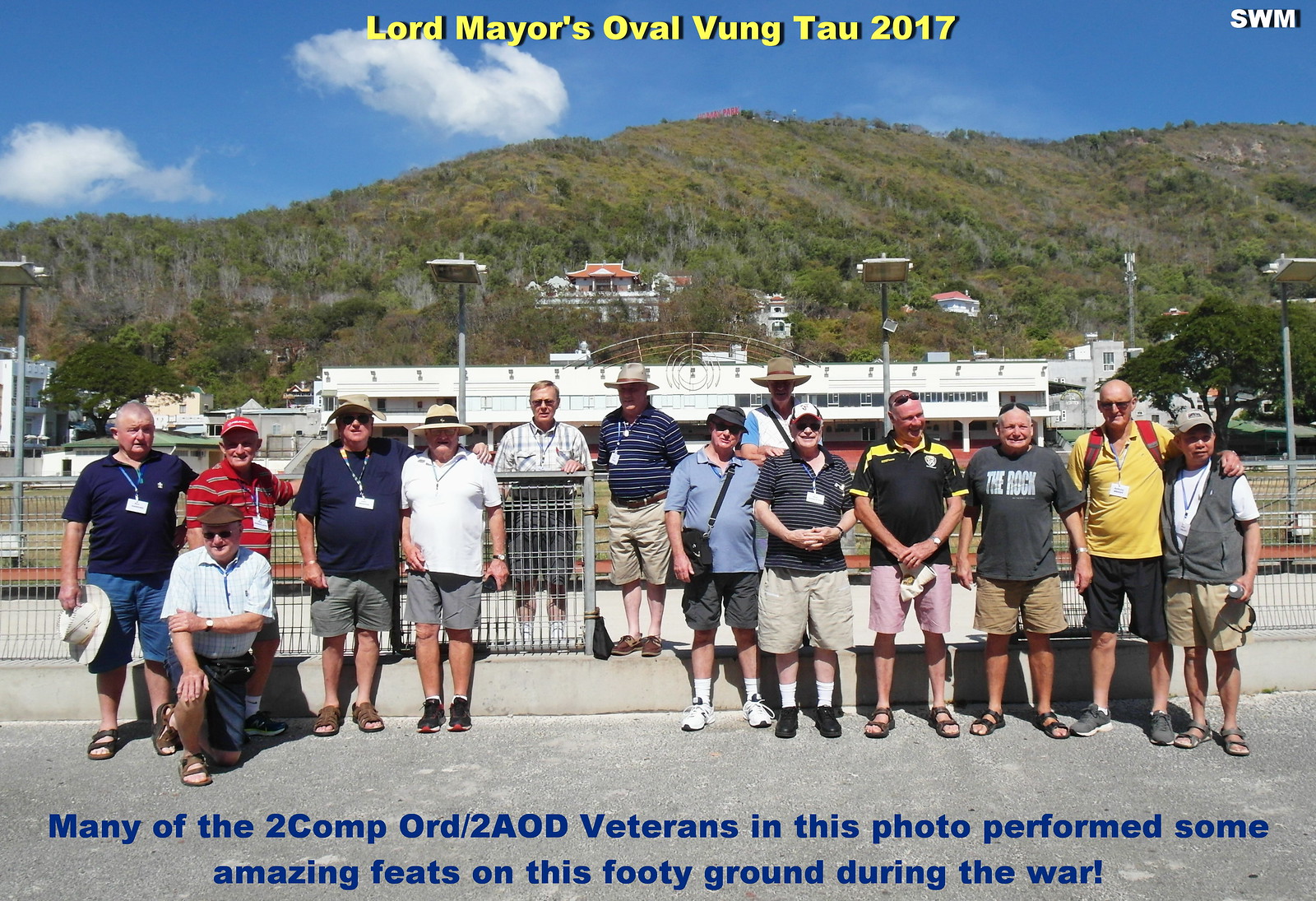A group photo features a gathering of over a dozen older gentlemen, ranging from their 40s to 60s, standing shoulder to shoulder and some with arms around each other on a cement sidewalk and parking lot. One man on the left is kneeling. They are dressed in various styles, including t-shirts, collared shirts, shorts, and hats, and most are looking directly at the center camera. The backdrop reveals a lush, grassy hillside adorned with sparse white houses with red tile roofs, partially obscured by greenery. Above the hillside, a partly cloudy sky fills the upper portion of the image. Yellow text at the top reads "Lord Mayor's Oval Vung Tau 2017," with "SWM" in white in the top right corner. Blue text at the bottom states, "Many of the 2 Comp ORD 2AOD veterans in this photo performed some amazing feats on this footy ground during the war." This indicates the group consists of veterans, photographed at the base of a mountain or large hill.